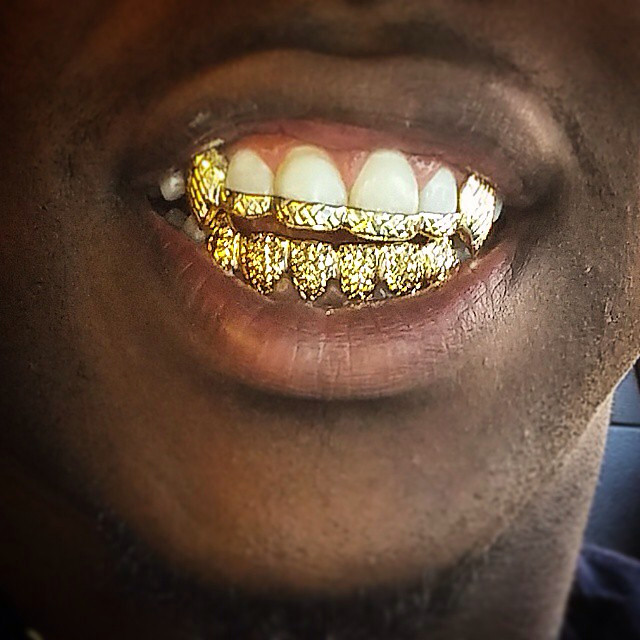This image depicts a very close-up, square-shaped photograph of a darker-skinned African-American man's mouth and lower face. He is smiling, displaying his teeth prominently. The man has a thin mustache on his upper lip, a slight goatee on his chin, and some five o'clock shadow stubble on his cheeks. 

The upper row of teeth includes canine teeth fully capped in shiny gold, whereas the four teeth in between (including the two front teeth and the two adjacent ones) feature gold caps on the lower half. The entire front bottom row of teeth is fully capped in gold. The gold on the bottom teeth appears textured, almost resembling diamond plating, giving it a very reflective and shimmery look. This intricate grillwork is a striking fashion statement, reminiscent of styles often seen among well-known rappers. Only the area from the chin to just above the upper lip is visible in the photograph.